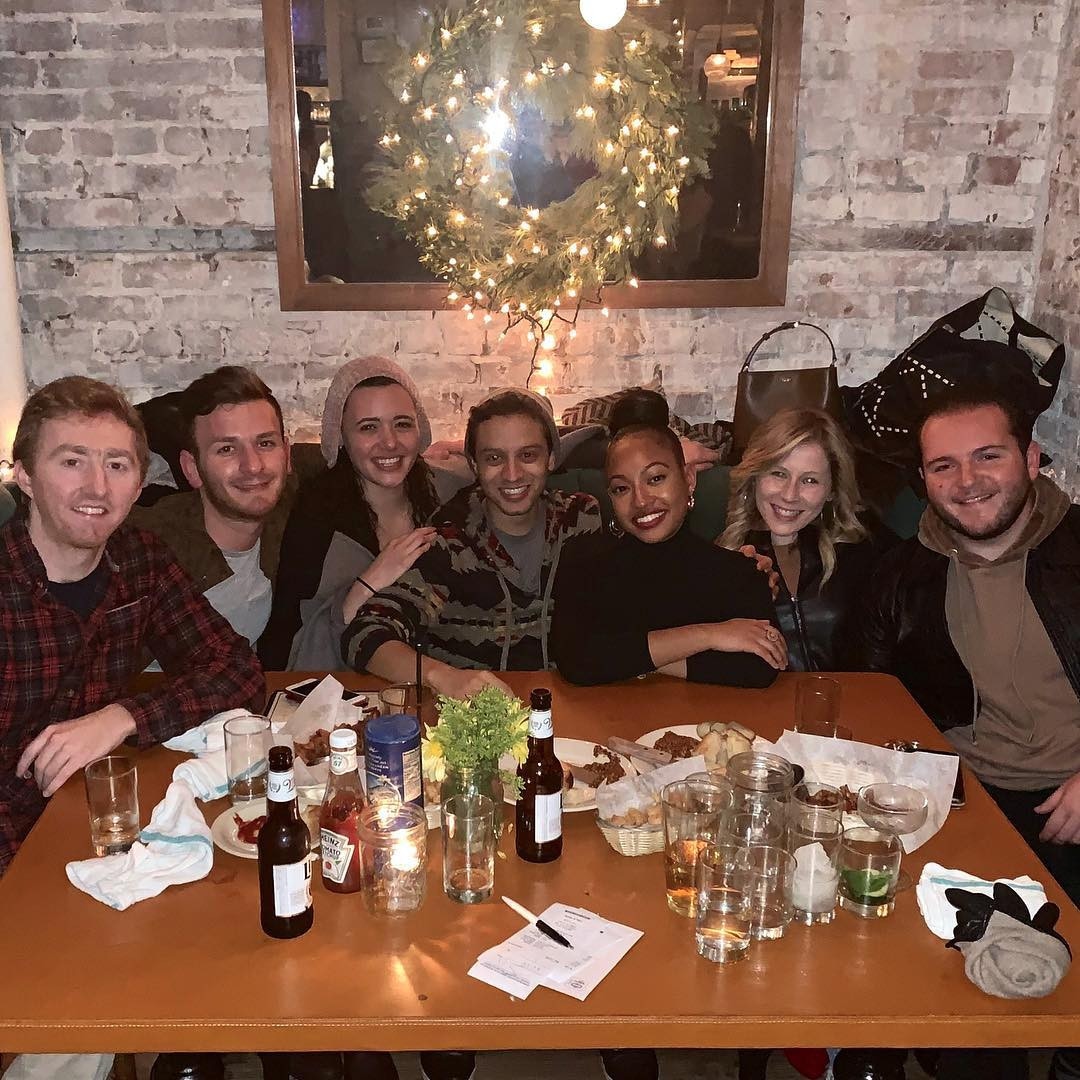This photograph captures a vibrant and joyful scene of seven young adults, appearing to be in their 20s or 30s, sitting around a square wooden table in what looks like a bar or restaurant. The group, a mix of four men and three women of various races, are arranged side by side, with two men on the far left, followed by a woman, another man, another woman, another woman, and a man on the far right. All seven are dressed in winter attire, with flannels, sweaters, and jackets, suggesting it's cold outside and aligning with the Christmas season indicated by the lit white wreath hanging on a rustic, whitewashed brick wall behind them. The table before them is cluttered with the remnants of their meal: empty beer bottles, glasses, soiled napkins, residue-covered plates, a bottle of ketchup, and a settled check with an ink pen on it. Their smiles and the natural, happy expressions on their faces suggest they've enjoyed their time together, making for a warm and festive scene.